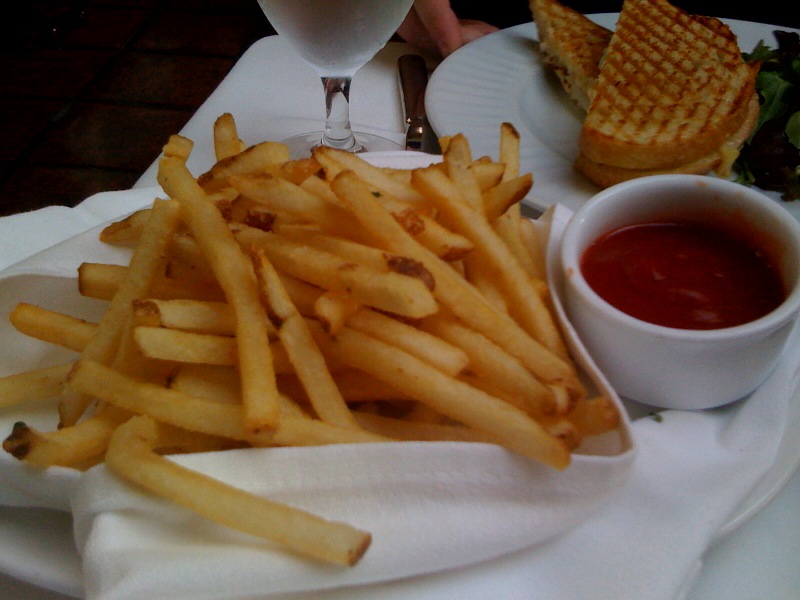The photograph depicts a meal arranged on a table, with the central focus being a generous portion of golden-brown French fries set atop a cloth napkin. To the immediate right of the fries, a small white porcelain bowl brimming with ketchup sits ready for dipping. Behind the fries, closer to the left, a tall glass goblet filled with water is visible, reflecting a cool transparency. In the top right corner, a white plate holds a panini-pressed sandwich accompanied by a serving of fresh greens, possibly lettuce or arugula. Just beyond the plate, a glimpse of a person's hand can be seen, suggesting the meal is being enjoyed in a relaxed setting, likely a restaurant. The colors in the image prominently feature warm golden browns, vibrant reds, lush greens, and the clean simplicity of see-through white elements, creating a visually appealing presentation of the meal.